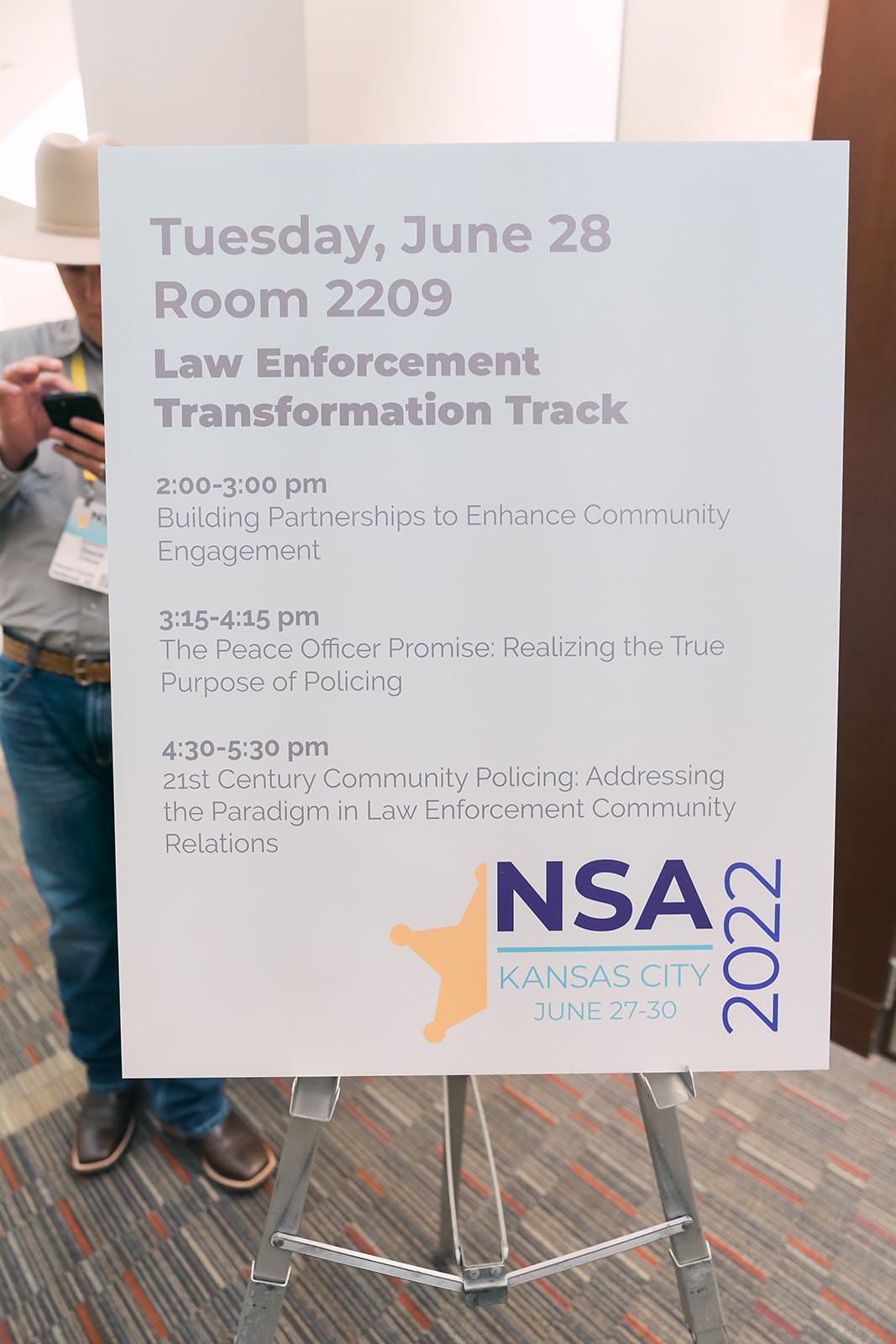The image features a large informational poster on a silver easel with visible legs connected by rods. The poster itself has a light gray background with darker gray and slightly lighter gray text. At the top left, it reads, "Tuesday, June 28th." Below that, it states, "Room 2209," followed by "Law Enforcement Transformation Track." The schedule on the poster includes: "2 to 3 p.m.: Building Partnerships to Enhance Community Engagement," "3:15 to 4:15 p.m.: The Peace Officer Promise: Realizing the True Purpose of Policing," and "4:30 to 5:30 p.m.: 21st Century Community Policing: Addressing the Paradigm in Law Enforcement Community Relations." In the bottom right corner, the poster displays "NSA" in large purplish-dark blue letters with a turquoise line and "Kansas City, June 27th - 30th, 2022," accompanied by half of a star-like badge. Standing behind the poster, partially visible, is a man wearing a white cowboy hat, a gray shirt, blue jeans, cowboy boots, and a brown leather belt. He also has a lanyard and is intently looking at his cell phone. The background includes a gray carpet with orange lines, a white wall, and a brown doorway to the right.